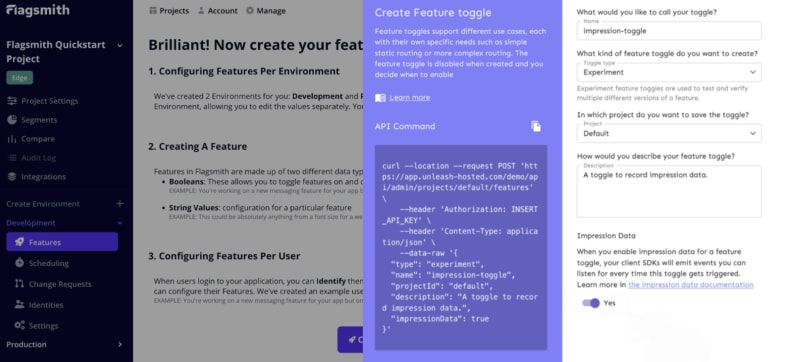This image showcases a demo or example of a web-based application, likely an interface for a feature management tool. The layout consists of two main sections: a program interface on the left and a sidebar menu on the right, separated by a narrow vertical white gap.

On the left, the screen is dominated by three vertically aligned, rectangular panels in a landscape orientation. The leftmost panel is dark blue, featuring "Flagsmith" in white text at the top, followed by "Flagsmith Quickstart Project," and a green clickable button. This section also includes clickable options like project settings, segments, and options for development and environment creation.

The middle panel, which is whitish-gray, provides three top tab options: "project," "account," and "manage." The header here reads "Brilliant, now you can create features," and offers three actions: configuring features per environment, creating a feature, and configuring features per user, each accompanied by a brief description.

The rightmost panel is light blue with white text that reads "Create Feature Toggle." Below this header, there's a brief description followed by an "API Command" section that contains a darker blue box with white coding text. Adjacent to this is a white input box prompting, "What would you like to call your toggle?" where users can enter a name and specify settings.

On the right side of the image, the sidebar menu supports easy navigation within the application, enhancing its user interface and functionality.